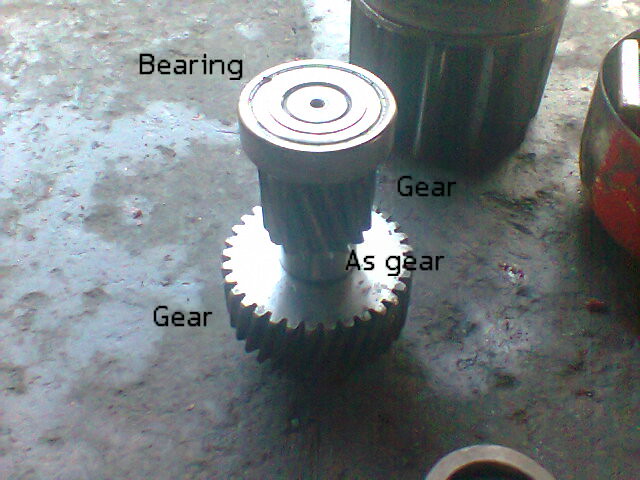The photograph displays a detailed close-up of mechanical components, primarily focusing on a thick, circular metal gear with jagged, toothed edges. The image is taken from an overhead perspective in what appears to be a workshop setting. The base of the gear rests on a slightly dirty, oil-stained concrete surface. Central to the composition is a large, smooth screw labeled "bearing" emerging from the middle of the gear. Rising from the gear is a cylindrical column, which transitions into another segment of gear, marked by a textured, arched, and jagged exterior pattern. This cylindrical column narrows towards the top. Text labels overlay the image, marking various components: "gear" on the bottom left and center, and "bearing" on the top left of the screw. There is natural light illuminating the scene from above, and additional metallic cylinders are visible in the top left corner of the image, enhancing the industrial atmosphere.